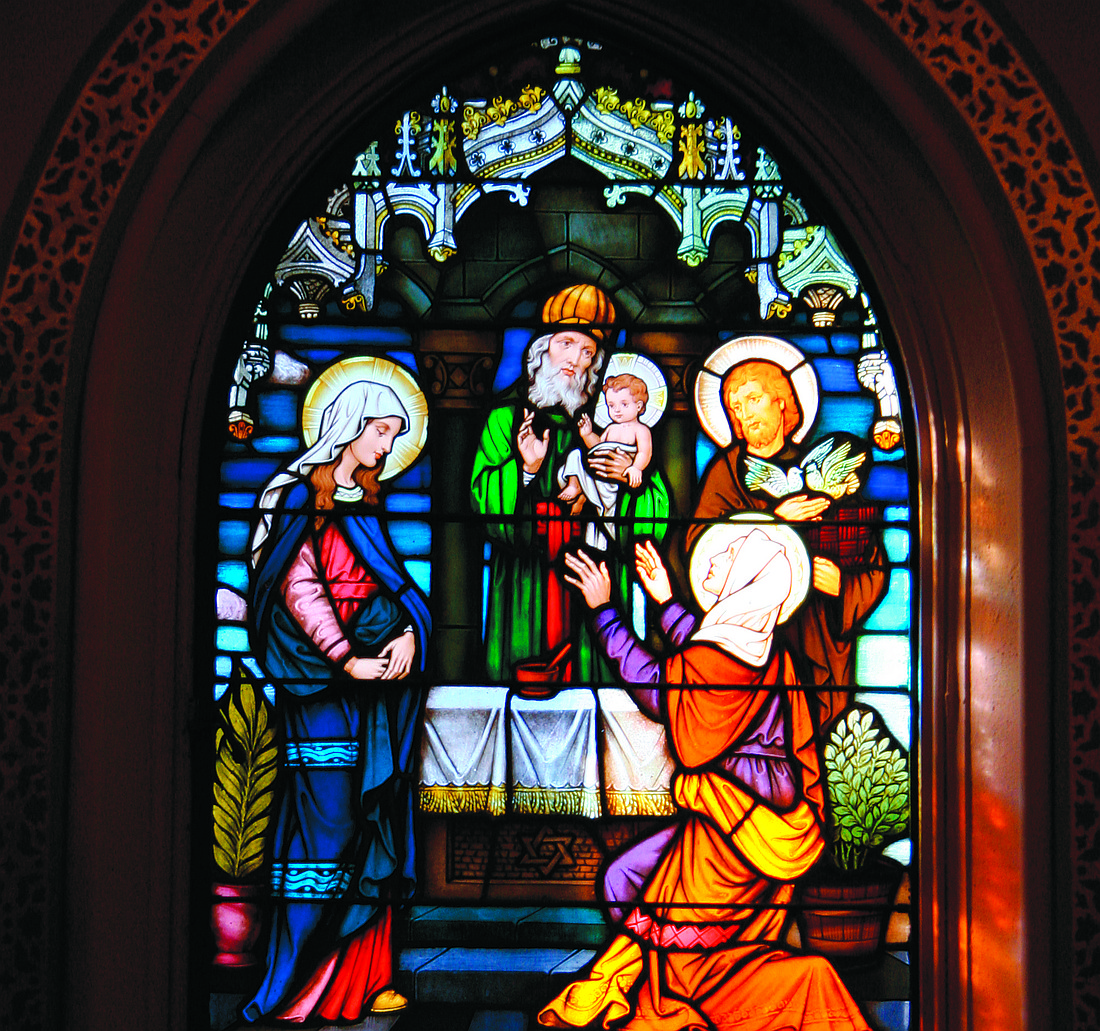The image depicts a detailed and vibrant stained glass window, likely located within a church. The centerpiece features an arched dark wood frame with gold metallic accents, encasing a biblical scene. The stained glass illustrates a notable religious tableau: at the center stands an older man with a white beard, adorned in a green robe and orange hat, holding an infant, presumably baby Jesus encircled by a halo. To the left, a woman, possibly Mary, dressed in blue with a white veil over her head, either appears pregnant or in a state of serene contemplation with her hands gently clasped. To the right, a kneeling woman in an orange and purple dress with a white cloak extends her hands up towards the child. Beside her, another man, likely Joseph, is depicted with an orangish beard, dressed in a brown robe, holding two doves. Additional elements such as an altar with a white cloth and vibrant ribbons at the top enhance the sacred atmosphere, while accents like green plants in pots and a vase contribute to the composition’s intricate design.